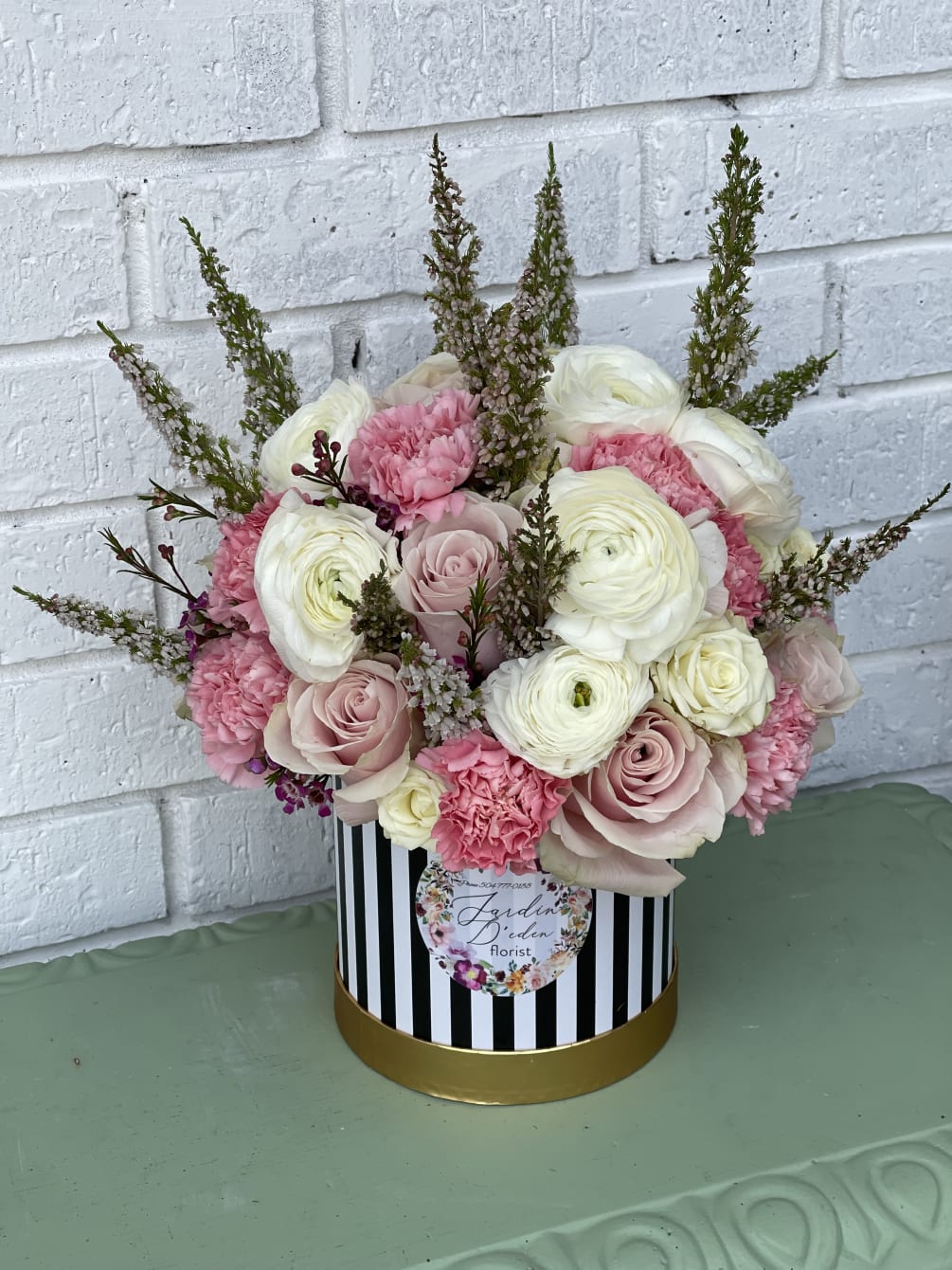This detailed photograph captures a beautifully arranged floral bouquet set against a white painted brick wall. The arrangement is displayed on a table with a light olive green surface, possibly made of masonry with decorative scrolling at the front. The floral centerpiece is held in a cylindrical container with a striking design: a gold base transitioning into black and white vertical stripes. A label on the container reads "Jardin d'Eden Florist," written in elegant cursive and adorned with a floral design, and includes the phone number 504-777-0655.

The bouquet itself is lush and overflowing, featuring an array of flowers in various shades of pink, white, and ivory. The assortment includes pink and mauve roses, white roses, white peonies, and possibly pink carnations. Interspersed among the blooms are sprigs of greenery and possibly some dried spiky plants or flowers, adding texture and height to the arrangement. The flowers vary in color from light pinks to darker pinks, yellow-tinged whites, and lilac hues, creating a vibrant and eye-catching display.